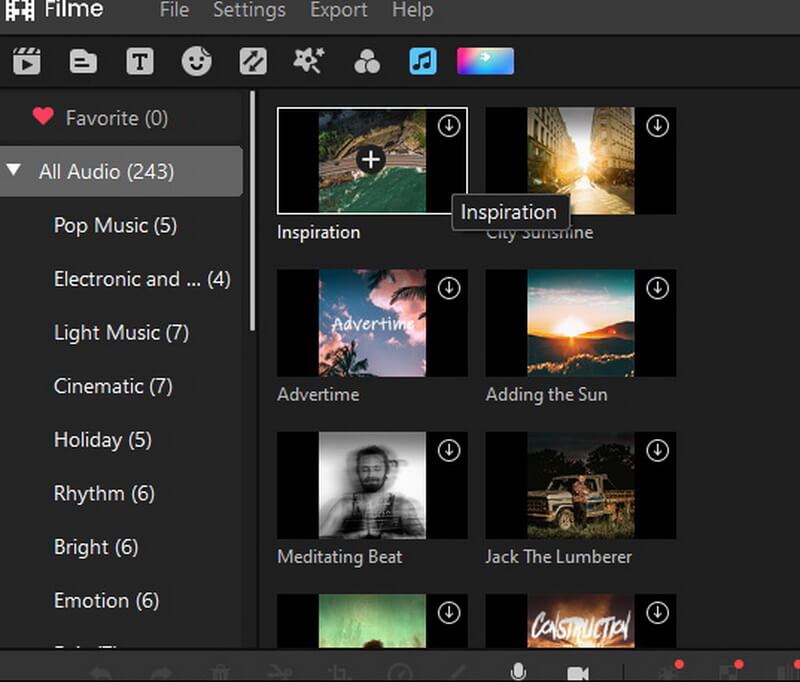Screenshot of a video editing software interface, featuring a sleek design with a grey navigation bar across the top. On the far left of the bar is a logo which includes the text "Filme" in white, accompanied by a filmstrip icon. Toward the right of the grey bar, four menu options are displayed: File, Settings, Export, and Help.

Below the top navigation bar is a secondary row of nine tool icons. These icons represent (from left to right): a video symbol, a folder, a text tool, a sticker tool, two diagonal arrows, a star, three overlapping circles, and a music note.

On the left side of the interface is a sidebar labeled "Favorite" at the top with a red heart icon next to it. Directly below this, a dropdown menu indicates "All Audio (243)," suggesting a collection of 243 audio files. Along both the left and right sides of the interface are panels displaying various themes, videos, and video thumbnails, providing additional options and resources for video editing.